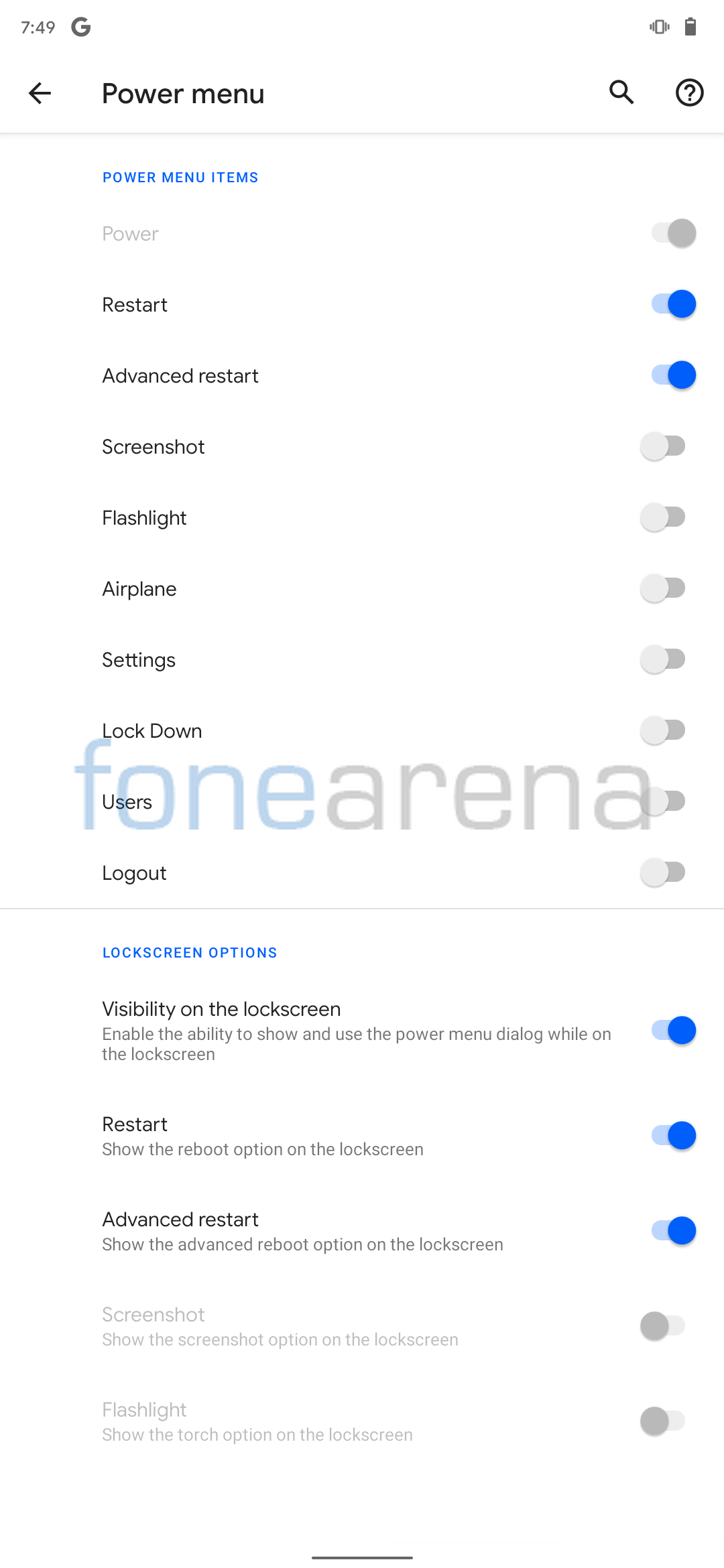This screenshot captures a specific subsection of an Android smartphone's power menu. In the top left-hand corner, the time is displayed as 7:49, although it's unclear whether this is a.m. or p.m. The Google logo appears, indicating the presence of Google software. In the top right-hand corner, the icons show that the phone is set to vibrate mode and the battery level is approximately 70%. 

The power menu, depicted in a white light color scheme with blue accents, lists various options. The choices for "Restart" and "Advanced Restart" are enabled, while other options, including "Screenshot," "Flashlight," "Airplane," "Settings," "Lockdown," "Users," and "Logout," are disabled. The "Power" option appears grayed out, suggesting it cannot be modified. Under the lock screen options at the bottom, "Visibility on Lock Screen" is enabled, while "Restart" and "Advanced Restart" remain active. The final two options are disabled, completing the menu's configuration.